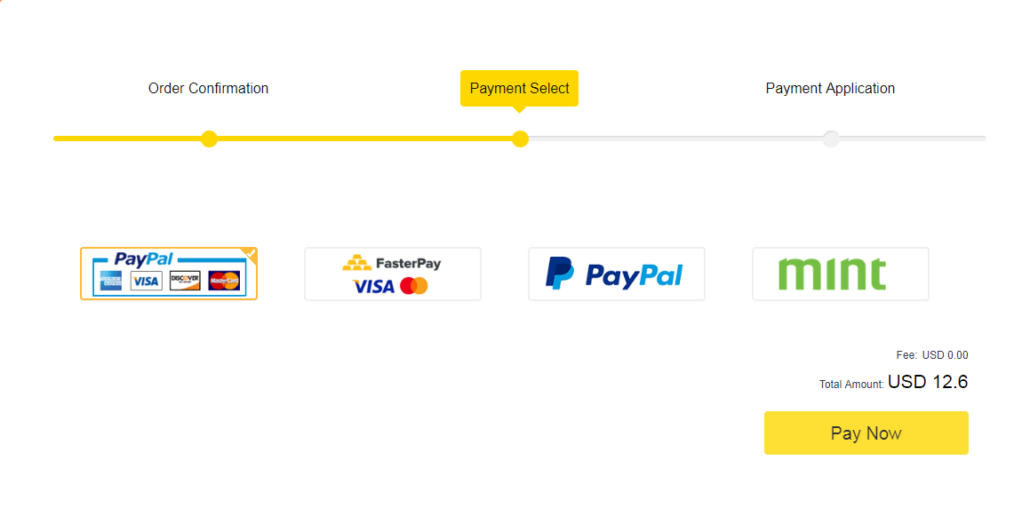This cropped screenshot captures the "Payment Select" screen from an online transaction process. At the top, the screen shows a three-step progress bar indicating the stages: 'Order Confirmation,' 'Payment Select,' and 'Payment Application.' A gray bar runs horizontally underneath these steps, featuring circular icons centered beneath each label. The left side of the bar (encompassing 'Order Confirmation' and 'Payment Select') is highlighted in yellow, while the bar stops at 'Payment Select,' which is also highlighted in yellow.

Beneath the progress bar is a horizontal list of payment options presented as small rectangular boxes. The first option, PayPal, is selected and displays very small square thumbnails of American Express, Visa, Discover, and MasterCard logos. To the right, the next option is FasterPay, accompanied by the Visa logo. Following that, there's a direct PayPal option without associated credit cards. The final option on the right is Mint.

At the bottom right of the screenshot, in small black font, it reads "Fee USD 0.00." Below this, the "Total Amount USD $12.60" is displayed. At the very bottom, a yellow button labeled "Pay Now" is prominently featured, inviting the user to proceed with the payment.